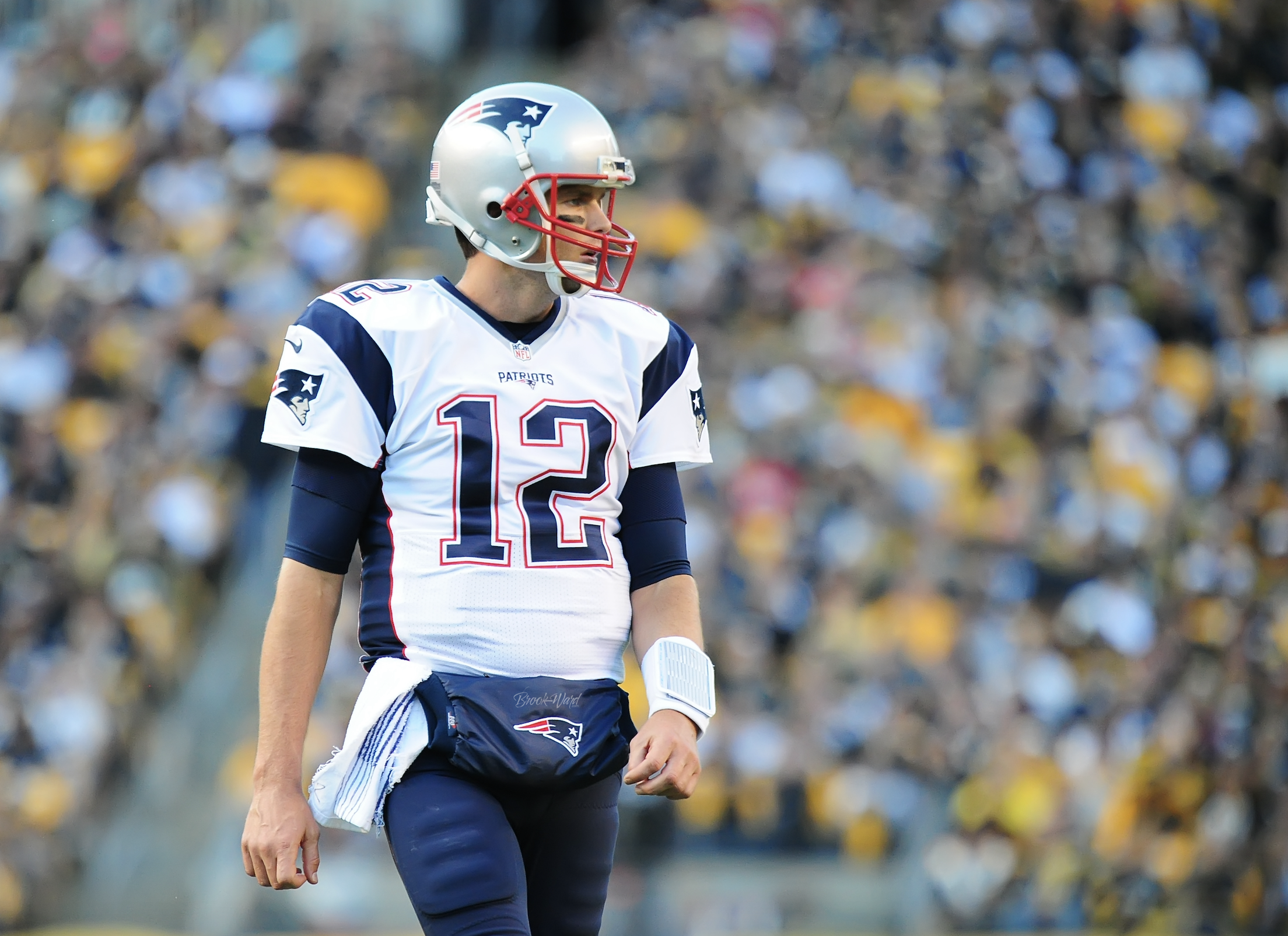This detailed photograph features Tom Brady, the celebrated New England Patriots quarterback, captured in a dynamic pose during a game. He is adorned in the iconic Patriots uniform, primarily white with blue accents. Prominently displayed on his chest, shoulders, and helmet is his number 12, highlighted by a red outline. The jersey is emblazoned with "Patriots" in blue text at the top, complemented by blue thigh pads and a silver helmet with a red front and the Patriots logo on each side.

On his left wrist, Brady sports a white wristband that doubles as a playbook. A striped towel hangs from his right hip. Additional equipment includes a fanny pack at the front of his blue pants, also bearing the "Patriots" inscription. The backdrop is a bustling stadium filled with a blurred sea of spectators, lending a sense of movement and intense focus as Brady glances to his left, seemingly mid-play. This image captures both the detailed elements of his gear and the larger atmosphere of an electrifying football game.